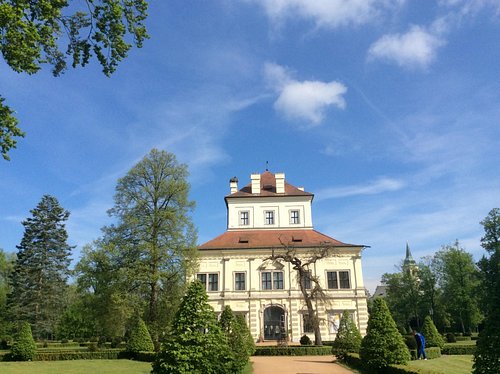This highly detailed and lifelike painting features an expansive, off-white mansion with a grand, ornamental front door. The majestic structure stands tall with two primary stories, a roof, and an additional smaller upper story crowned by three prominent chimneys. The impressive residence is fronted by a wide, meticulously laid concrete driveway that leads up to the house. Along the driveway, perfectly pruned trees shaped like Christmas trees line the path, adding to the regal aesthetic. Surrounding the property, well-maintained boxwood hedges and flourishing shrubs add vibrant greenery. The backdrop of the painting showcases a serene sky, painted with delicate wisps of clouds against a blue expanse. In the foreground, a figure dressed in blue can be seen from a distance, adding a touch of human presence to the otherwise tranquil and picturesque scene.